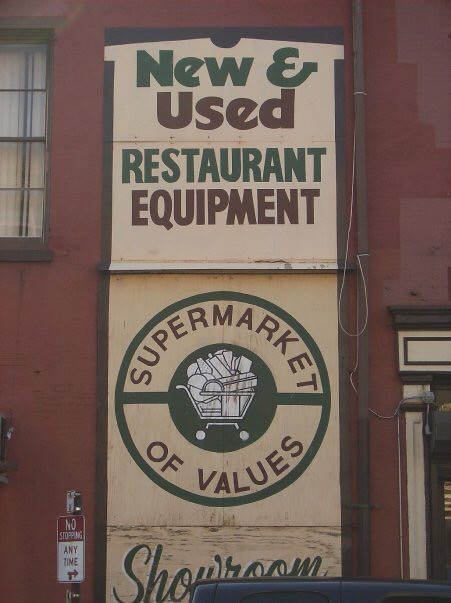This photograph, captured outside a restaurant, features a prominent red brick wall adorned with black-bordered windows that have white shades. In the top left corner of the image, part of the building is cut off, while the bottom right corner shows a door with black and white trim. The focal point is a vertically oriented, rectangular store sign that extends up the height of the building. The sign has a beige background with black bordering, displaying the text "New and Used Restaurant Equipment" in bold green and black letters. Additionally, there is a circular logo on the sign. The top arc of the logo reads "Supermarket" in blackish-red text, and the phrase "of Values" is situated underneath, followed by another line of text beneath that, although it is unclear in the image. This detailed and descriptive caption paints a vivid picture of the scene for the viewer.